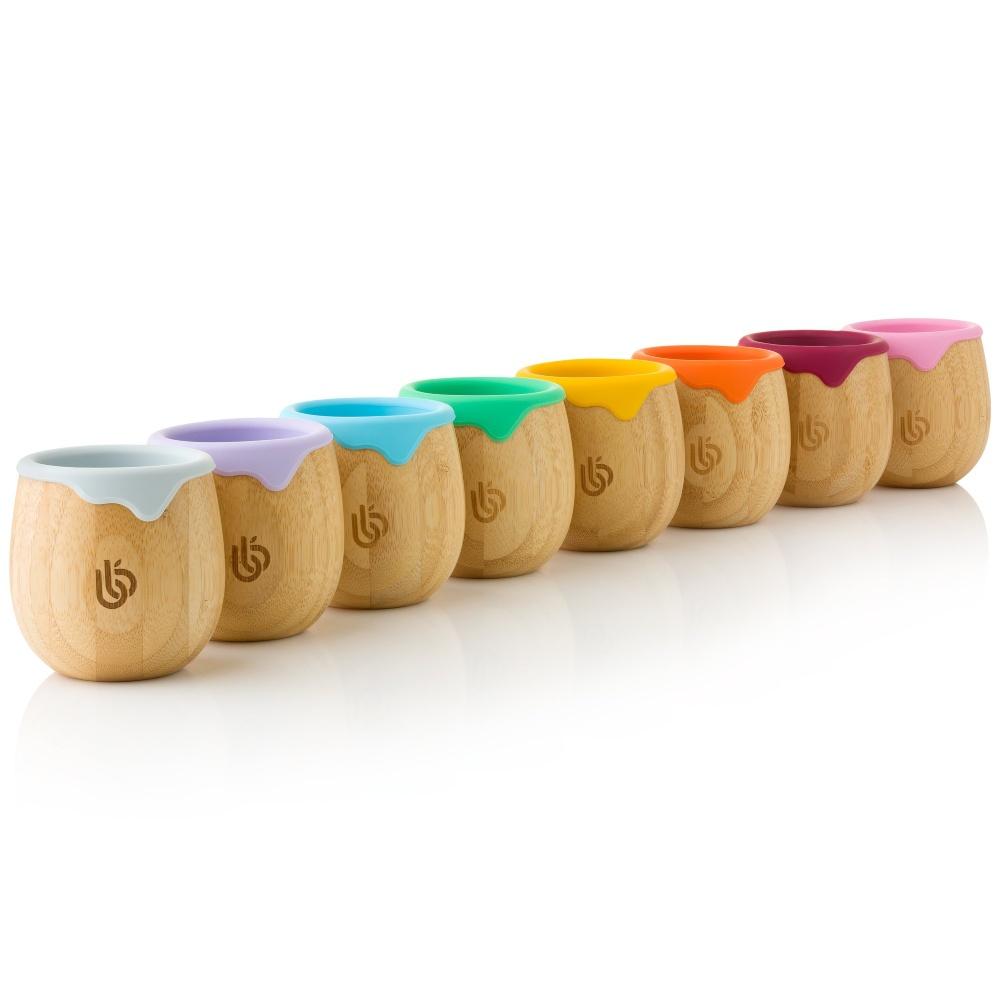The image showcases a lineup of eight small, untreated wooden jars arranged diagonally against a pristine white background, giving a sleek and minimal aesthetic. Each cylindrical jar, resembling miniature honey pots or baby food containers, features an intricate, engraved company logo on the front—two interlocking lowercase 'b's, designed to evoke the look of a tree with a leaf detail. The jars are capped with silicone lids that appear to drip like paint, adding a splash of color to the rustic wood. These lids come in a spectrum of hues from left to right: white, lavender, light blue, mint green, mustard yellow, orange, maroon-purple, and light dusty pink. The reflection of the jars on the glossy white surface beneath them adds an elegant touch to the overall composition. The lids' designs and the vivid colors give the impression of paints inside each jar, enhancing the visual appeal of this beautifully arranged display.